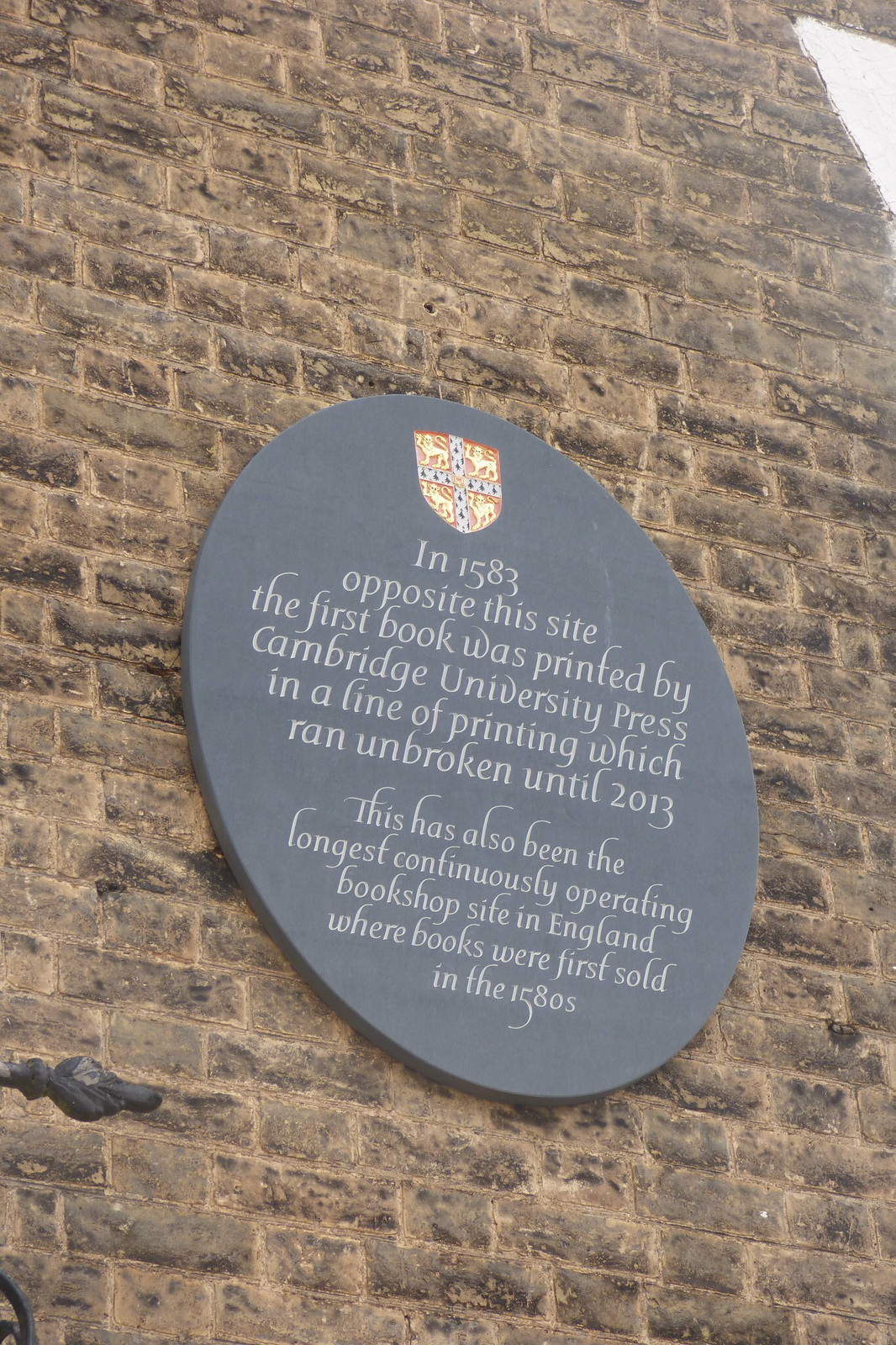The image features a prominently displayed plaque mounted on a dark brick wall, which occupies the entirety of the background. The plaque, centrally positioned, bears a shield or coat of arms at its top. The text on the plaque, written in white, reads, "In 1583, opposite this site, the first book was printed by Cambridge University Press in a line of printing which ran unbroken until 2013. This has also been the longest continuously operating bookshop site in England where books were first sold in the 1580s." The scene appears to be set outdoors in daylight, likely near a historic bookstore dating back to the 1500s. The predominant colors in the image are shades of tan, black, gray, white, yellow, and orange.